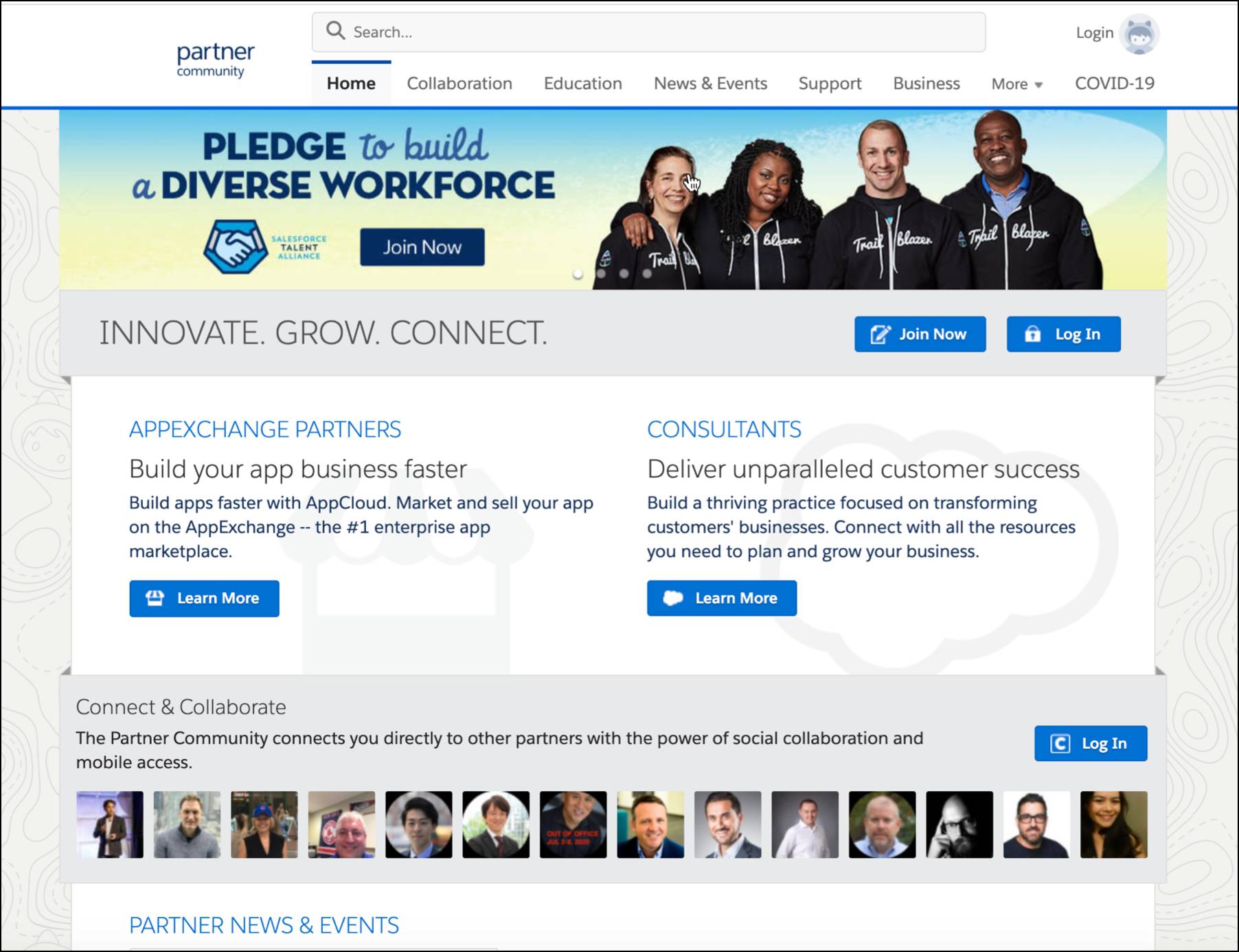At the top of the website, there is a white navigation menu containing the website's name and its partner community on the left. In the center, a search bar is prominently placed, and to the right, a login button is easily accessible. The top menu navigation includes options for "Home," "Collaboration," "Education," "News and Events," "Support," "Business," "More" with a dropdown area, and "COVID-19." Above this menu, a banner features four individuals standing side by side, all wearing matching hoodies with the word "Trailblazer" emblazoned on them. The group consists of two women and two men: a white woman, a black woman, a white man, and a black man. To the left of the group, the banner prominently displays the message, "Pledge to build a diverse workforce." Below the banner, there are two rectangular blue buttons: one on the left that says "Join Now" and one on the right that says "Login."